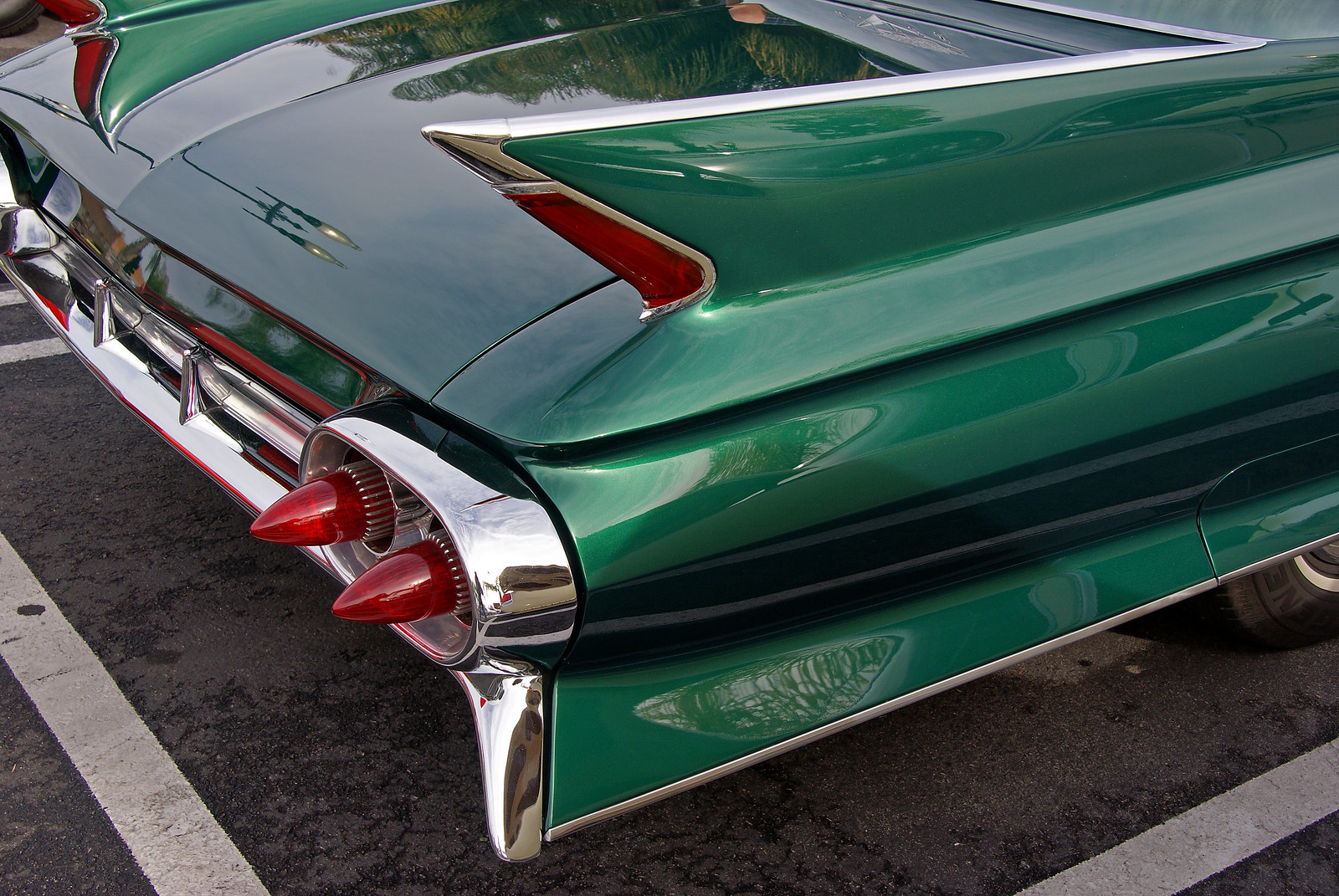This photograph captures the sleek, polished back side of a vintage, emerald green car, exuding the unmistakable elegance of a 1950s luxury vehicle. The car is positioned in an empty parking lot marked by white lines delineating the various parking spots on the black asphalt surface. The lighting reveals a clear daylight setting, further enhancing the car’s lustrous finish. The vehicle features highly polished steel bumpers and distinctive, cone-shaped red taillights, with two prominently visible due to the image's angle. On one side, a black rubber wheel adorned with a white stripe and silver rims stands out, emphasizing the car's classic, stylish design. The overall scene is void of any distractions, allowing the viewer to focus solely on the timeless beauty of this meticulously maintained automobile.